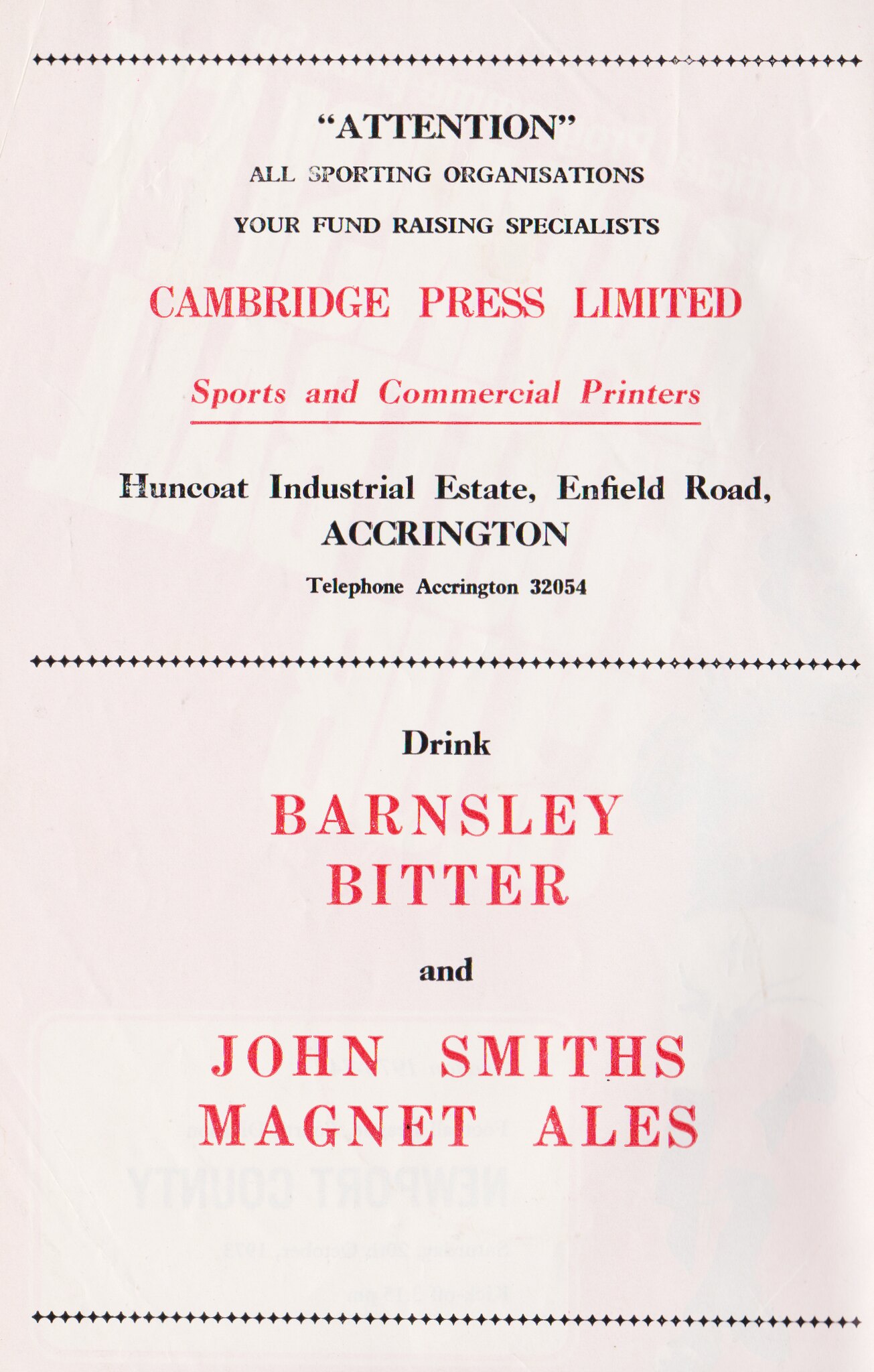The image is a photo of a slightly crinkled white piece of paper featuring a mixed advertisement or announcement in black and red text. At the very top, a line of black diamonds serves as a decorative header. Below this, in bold black text, it reads: "Attention, all sporting organizations, your fundraising specialists." This is followed by the name "Cambridge Press Limited" in striking red text, indicating their services as sports and commercial printers. Next, in black text again, it lists the address: "Huncote Industrial Estate, Enfield Road, Accrington," accompanied by the telephone number: "Accrington 32054." Another decorative line of black diamonds breaks up the sections. Below this, the word "drink" appears in black, leading into the names of beverages: "Barnsley Bitter" and "John Smith's Magnet Ales," both highlighted in red. The document is concluded with a final line of black diamonds at the bottom.